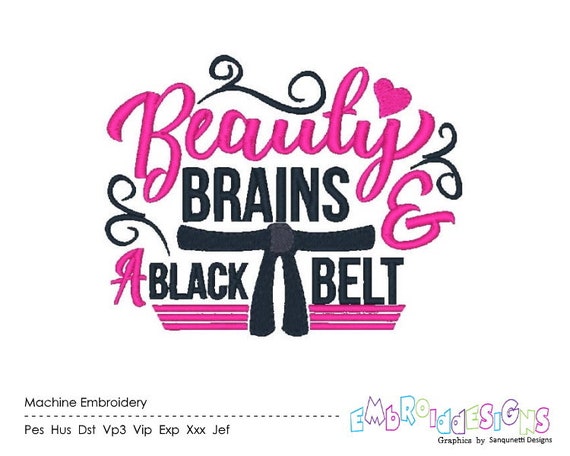The image features a logo on a predominantly white background. The centerpiece of the logo is a visually striking combination of text and design elements. Across the middle, "beauty" is written in bright pink cursive letters, surrounded by wispy lines in very dark purple or navy blue. Below this, in bold black letters, it reads "brains, and a black belt." A karate black belt is artfully integrated into this text, with two sashes hanging down. 

Beneath the main logo, in smaller text, it says: "machine embroidery" on the left side and "Embroidery Designs" on the right side, both printed in colorful letters. Additionally, technical embroidery file formats listed underneath include: PES, HUS, DST, VP3, VIP, EXP, XXX, JEF, with the text “Graphics by Sangwent Designs” appearing as well.